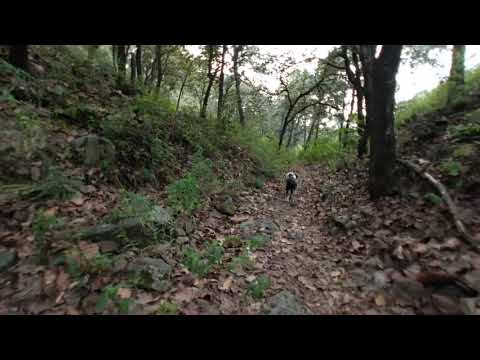In this daytime scene, set during a cloudy and hazy fall, a person is captured hiking through a dense, leaf-strewn forest. Positioned slightly right of center, they walk amidst a flurry of brown leaves and green patches of vegetation carpeting the forest floor. The backdrop showcases stately tree trunks, with one prominent trunk situated on the upper right side of the image. Overexposed light filters through the verdant tree branches, adding a subtle glow to the scene. Both the photographer and the subject appear to be navigating a gentle ravine, emphasized by the angle of the vegetation lining the hill. The image is framed by horizontal black bars at the top and bottom, giving it a cinematic quality.